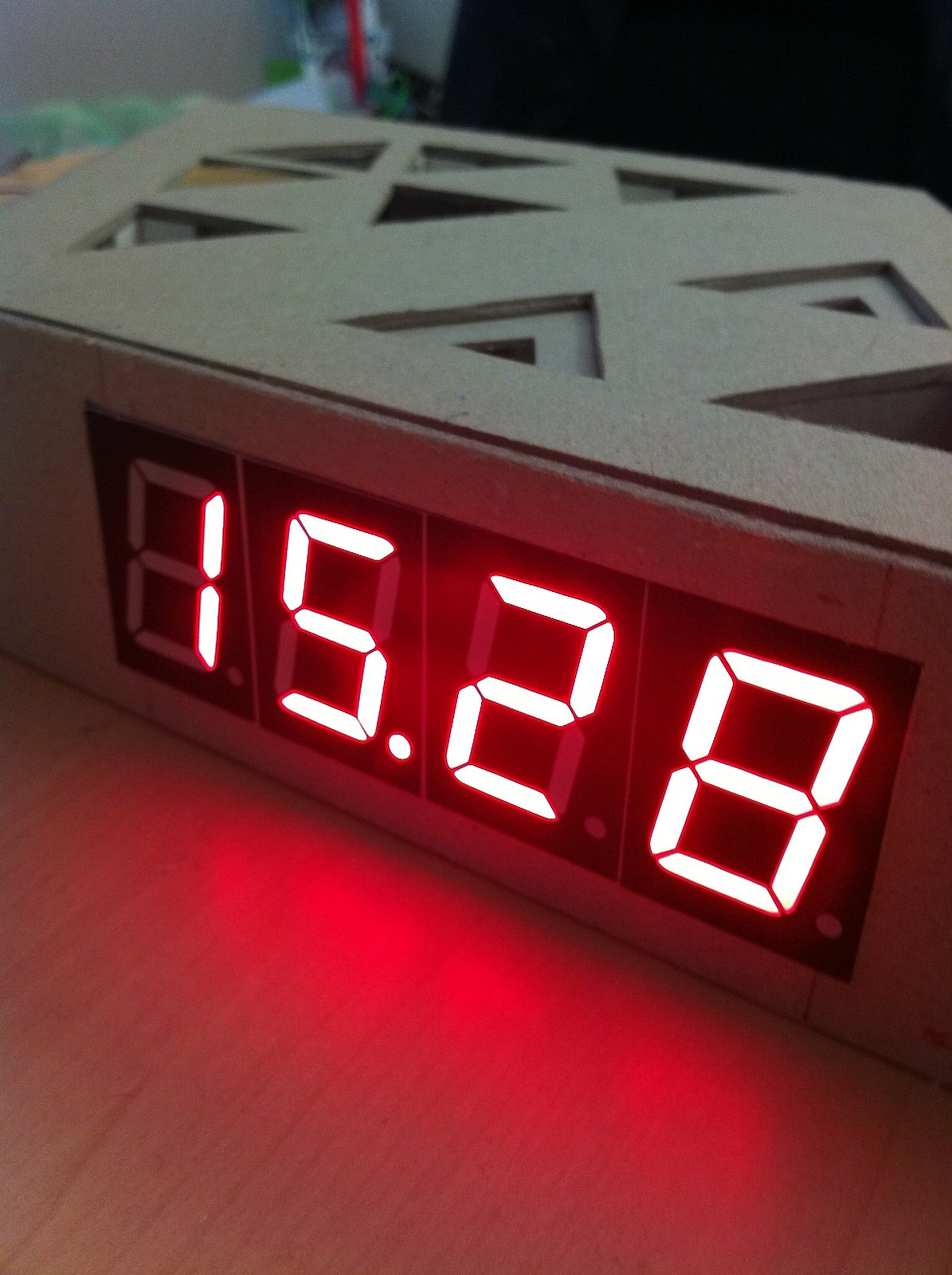This is a detailed color photograph of a unique digital clock. The clock is predominantly gray with a flat top, and its body angles down and faces to the left. It features a series of triangular cutouts along the top edges, with nine distinct triangular shapes pointing in various directions. These cutouts are complemented by a solid line running through the center of the top. The digital display, located on the side, is divided into four segments, each showcasing a portion of the time in white numbers outlined in red, creating a slightly red appearance. The displayed time reads 15:28. The glowing red numbers reflect vividly onto the light wooden surface below, which resembles a beige countertop or tabletop. Overall, the clock’s geometric design, with its triangular cutouts and glow, casts an eye-catching and somewhat mysterious aesthetic in the photograph.